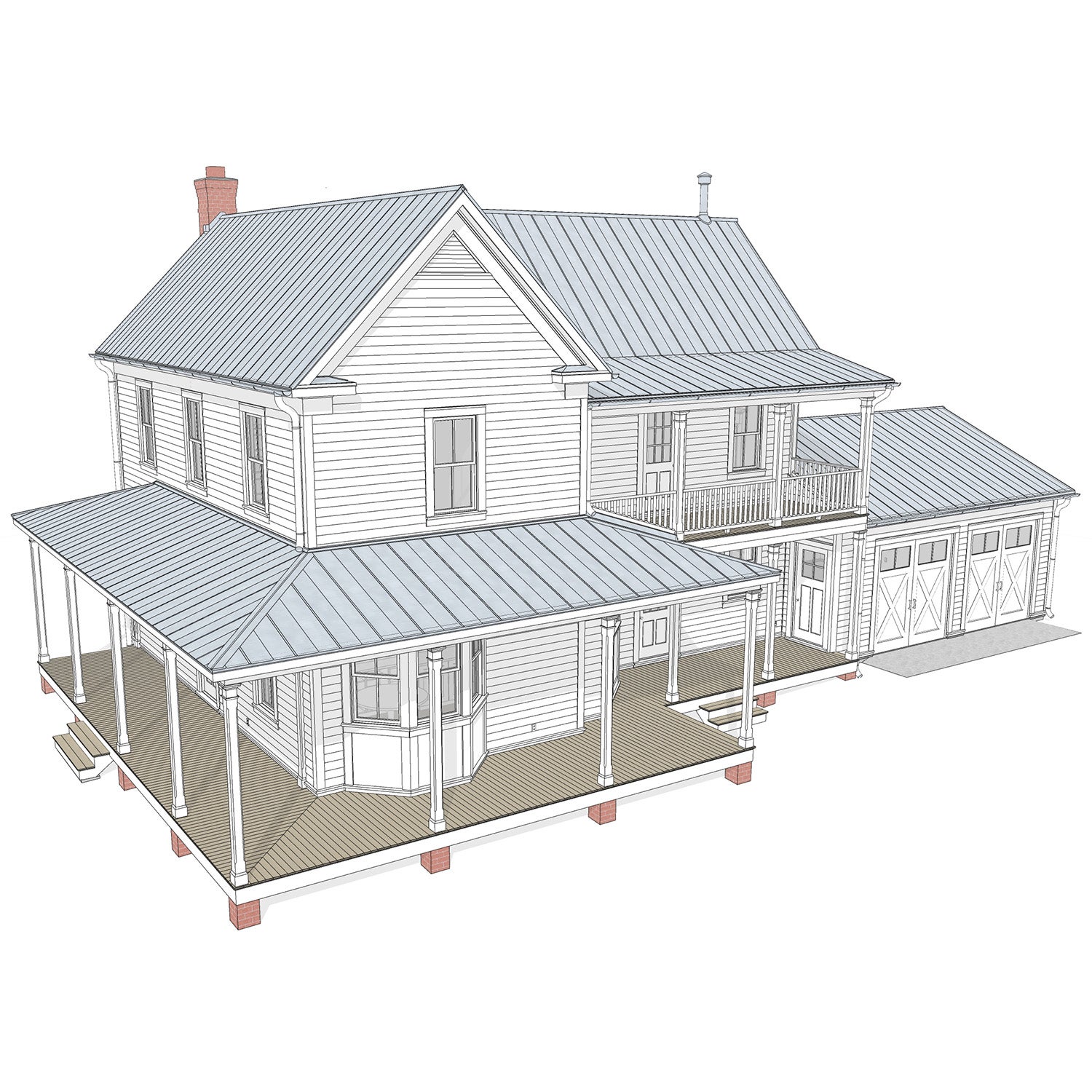This is an architect's elevation drawing of a large, two-story house. The house features a distinct design with two wings forming a 90-degree angle and an attached two-car garage at the rear. The exterior is predominantly white with accents of bluish gray, pale brown, and faded brick red. The structure has a wraparound veranda with a brown floor, supported by short, squat brick pillars, and a second-floor balcony with a wooden banister. The roof, which appears to be made of aluminum or light blue panels, includes a prominent rear chimney in a faded red hue. Numerous windows adorn the facade, including several bay windows on the ground floor. The overall appearance suggests a spacious, country-style home, well-suited for a rural or expansive setting.